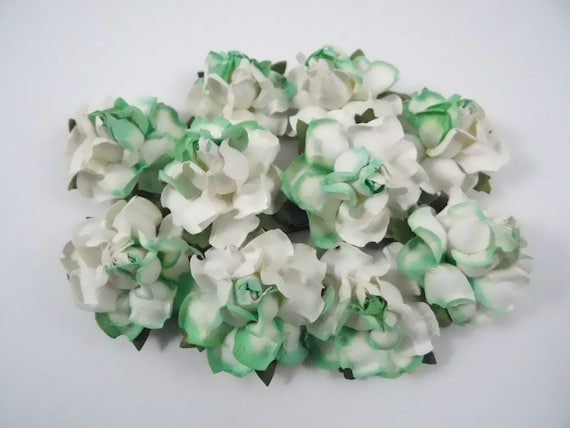The image depicts a cluster of ethereal, digitally enhanced flowers against a pristine white background. The flowers, which appear to be Photoshopped, are predominantly white with delicate, dainty petals. Each petal is uniquely edged in a leprechaun mint green, a hue uncommon in the natural world, accentuating their otherworldly appearance. The flowers are arranged in a circular formation, slightly lopsided, with a few central blooms encircled by others. Darker leaves emerge, particularly near the bottom, providing contrast to the lighter tones of the flowers. Small buds at the center of each flower add to the intricate details of this visually striking composition.